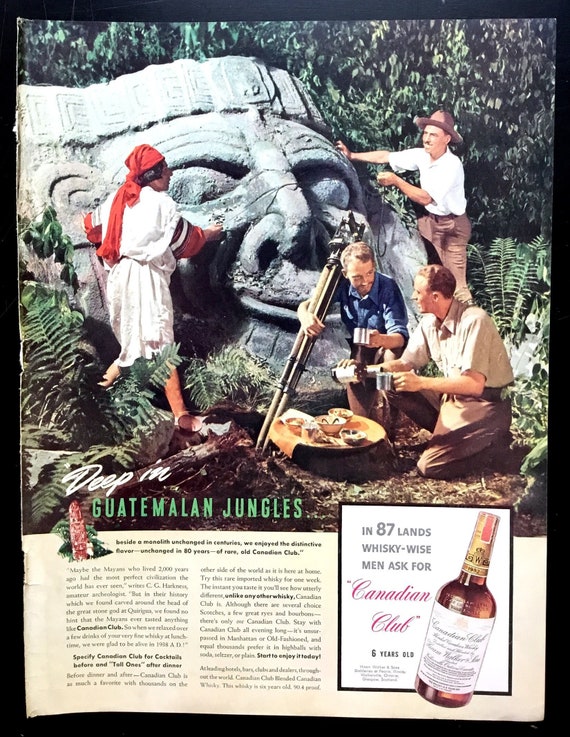This image is a vintage advertisement, likely from the 60s, featuring an archaeological expedition deep in the Guatemalan jungle. At the very top of the image, four men—three white and one dark-skinned—are uncovering a massive stone head, potentially from the Mayan era. Two men, one wearing a red headband and dressed in white, and the other with a hat, are kneeling in front of the ancient artifact and smiling. Another man holds a long tripod stand, while the fourth pours himself a drink from a bottle. There is a tree stump with bowls of food next to them. Text beneath the image reads, "Deep in the Guatemalan jungle," complemented by an inset picture of a Canadian Club whiskey bottle with text stating, "In 87 lands, whiskey-wise men ask for Canadian Club whiskey that’s five years old." The bottom third of the image has what appears to be a continuation of a magazine article, adding to the nostalgic and adventurous aura of the ad.